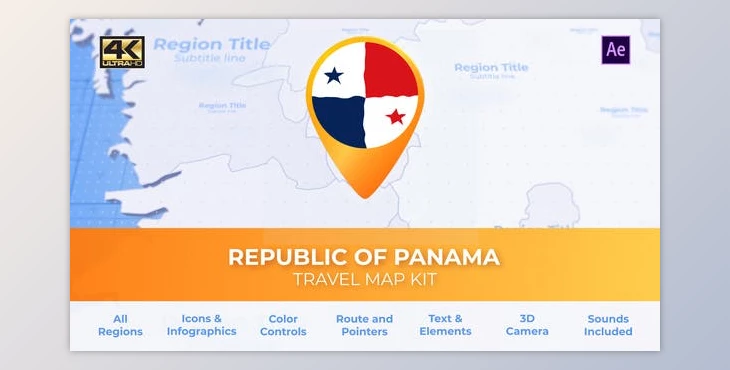The image depicts a comprehensive travel map kit for the Republic of Panama. The title prominently reads "Republic of Panama" with a subtitle line under the region title. The cover features the national flag of Panama presented in a circular form that tapers to a point. Positioned in the top right corner, there is a rectangular purple box housing a large "A" and a smaller "a." 

An orange strip fades to light orange and transitions to yellow as it extends from left to right. Below the title "Republic of Panama Travel Map Kit," the image highlights various features one can interact with, including all regions, icons and infographics, color controls, routes and pointers, text elements, 3D camera options, and included sounds. 

The map simplifies navigation and visualization, showing land areas in white and seas in blue on the left. The design appears textured and somewhat boxy, enhancing its practical layout for planning travel routes within Panama—especially beneficial for first-time visitors.